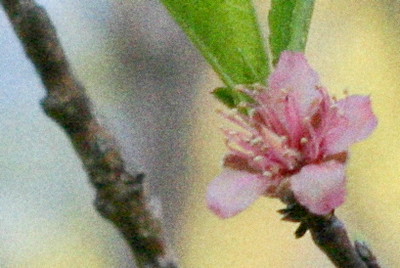The image captures a detailed, zoomed-in view of a vibrant pink flower blooming from a small branch on the right side of the frame. The flower features pale pink petals with darker pink tips and center, surrounded by finger-like protrusions that bear pollen-producing tips. Two green leaves are visible behind the flower, contributing to the intricate details of the scene. On the left side, there is another, bare branch with no leaves. The background is out-of-focus, creating a gradient that includes pastel yellows, light blues, tans, beiges, and some grayish tones, giving the image a nostalgic, slightly grainy appearance that enhances its delicate beauty. The overall composition emphasizes the intricate details and colors of the blooming pink flower and its immediate surroundings.